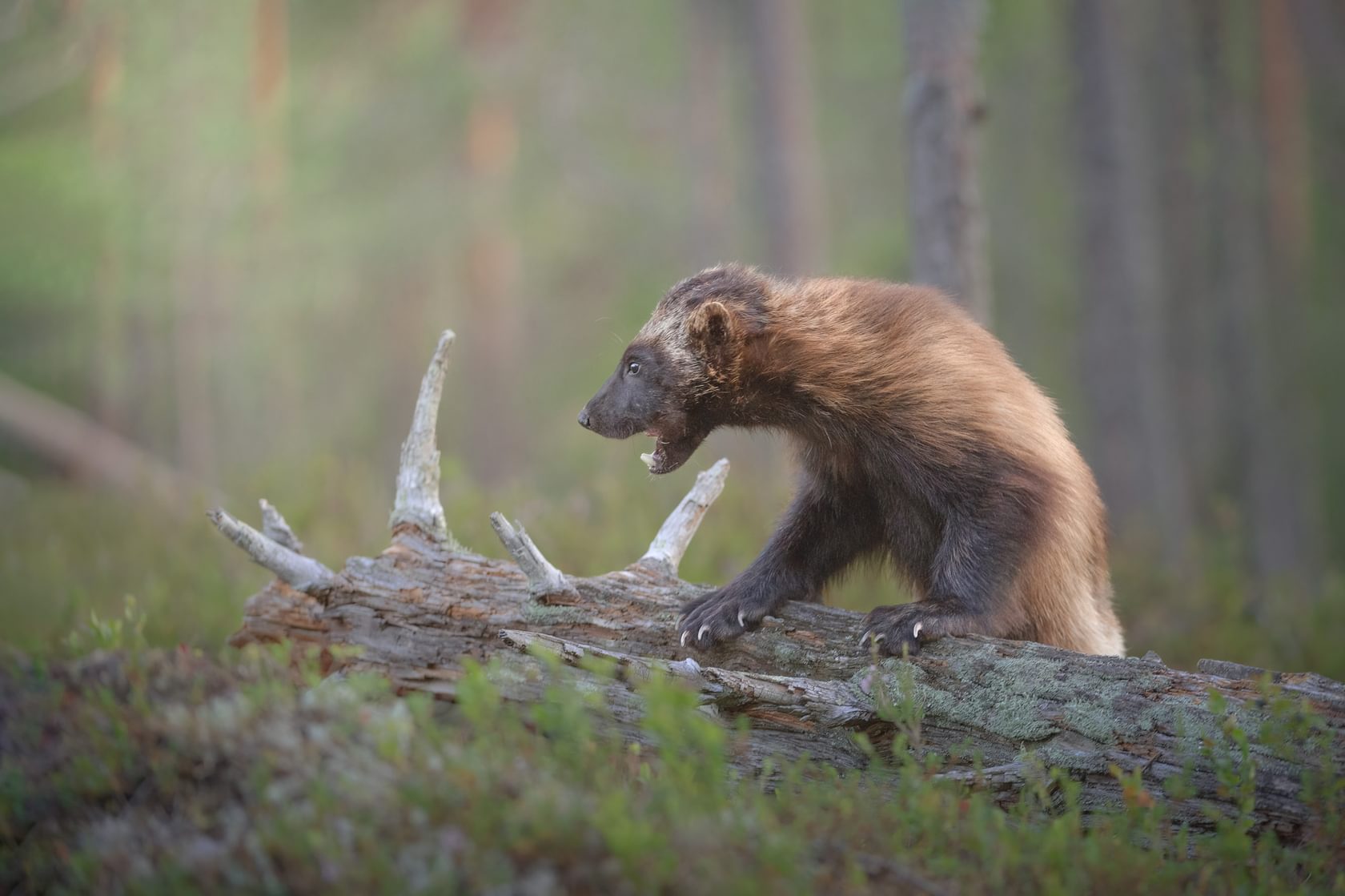The image features a young wolverine perched on a fallen tree stump in a dense forest setting. The wolverine has dark brown fur around its head, chest, and paws, with lighter fur towards its back. Its front paws rest on the log, revealing long, white claws. The animal's mouth is open, showing its teeth and giving the impression that it might be growling or calling out. Its body language appears focused and somewhat menacing, with its head turned slightly to the left and one eye visible. The wolverine has a black and brown coloration, with black fur around its eyes and nose, and a mix of black and brown across its body. The background consists of tall, thin trees and blurred vegetation, enhancing the sharp focus on the young wolverine, which appears to dominate the middle ground of the image.